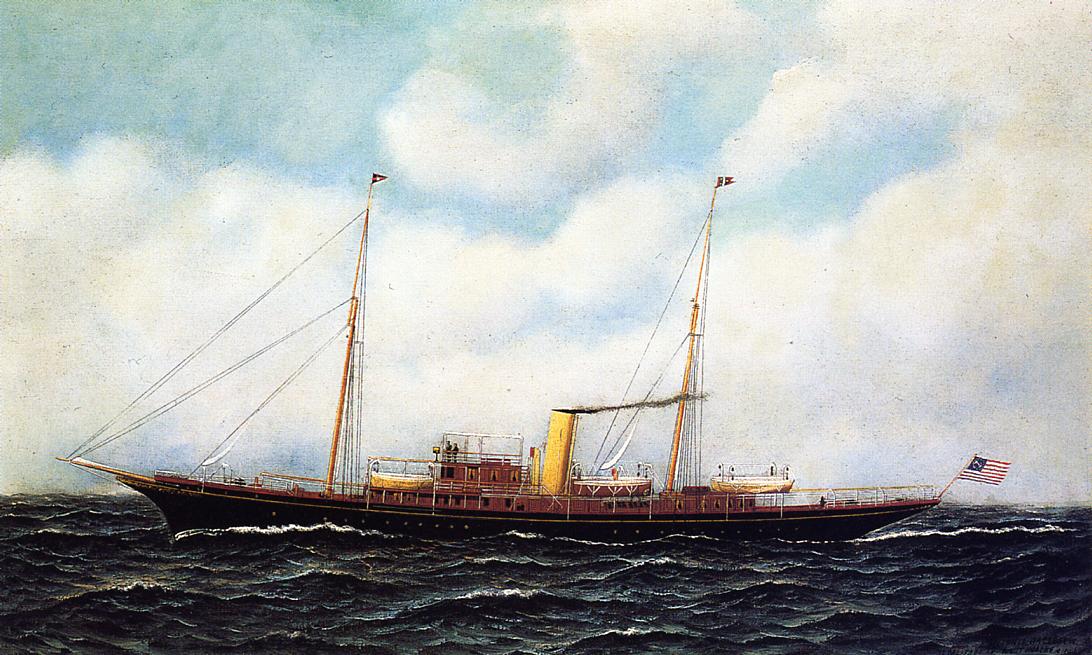This horizontal rectangular image portrays an old ship at sea, possibly a painting from over a hundred years ago. The vessel is long and sits low in the water, devoid of visible sails on its wooden masts, suggesting it has some form of power. At the stern, an American flag with red and white stripes and a blue area—with unclear stars—flutters in the wind. The center of the ship features a yellow smokestack emitting black smoke, with guardrails also visible. The sky is a mix of fluffy white clouds and patches of blue, while the dark, choppy sea below, with white-capped waves, indicates rough conditions.